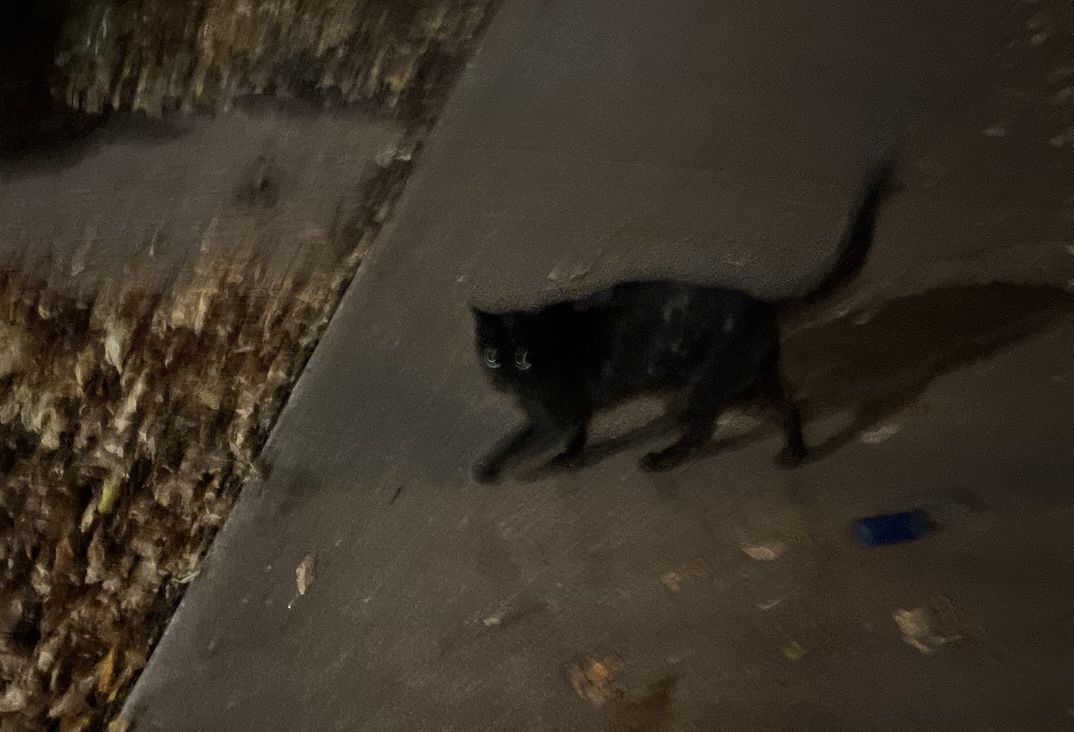This photograph captures a nighttime scene featuring a small black cat on a dimly lit sidewalk. The image is notably blurry, making it challenging to discern fine details. The cat's green eyes stand out amidst the blur, reflecting the nightlight that illuminates the entire scene and casts a shadow of the cat. Adjacent to the cat lies an indistinct, blue item that may be a cell phone. Surrounding the cat are what could be dead leaves or a patch of brown rocks, adding to the nocturnal ambiance. The sidewalk itself appears dark, possibly a tan hue obscured by the low light. The overall impression is of a fleeting, hurried moment, perhaps as a person quickly snapped a photo of the cat, which seems somewhat apprehensive in its posture.